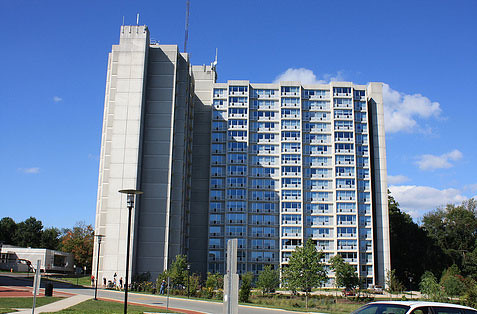This full-color outdoor photograph captures a bright, mostly sunny day with a vivid blue sky adorned by a few low-hanging cumulus clouds. Dominating the image is an 18 to 20-story high-rise apartment building that is primarily white and gray and features walkout balconies on its front side. The building is flanked by several trees, and greenery, including grass and bushes, is visible in front of it. In the lower right-hand corner, the hood of a white car is partially cut off. 
A street runs in front of the building, separated by a grassy area with some trees, a black garbage can, and a walking path. Several white signposts and lampposts are also visible. On the far left of the photograph, there is a shorter, trailer-like white building, possibly an office. The scene includes a couple of people, possibly three, riding their bikes along the road, and the presence of someone standing in front of the apartment building can be vaguely discerned.